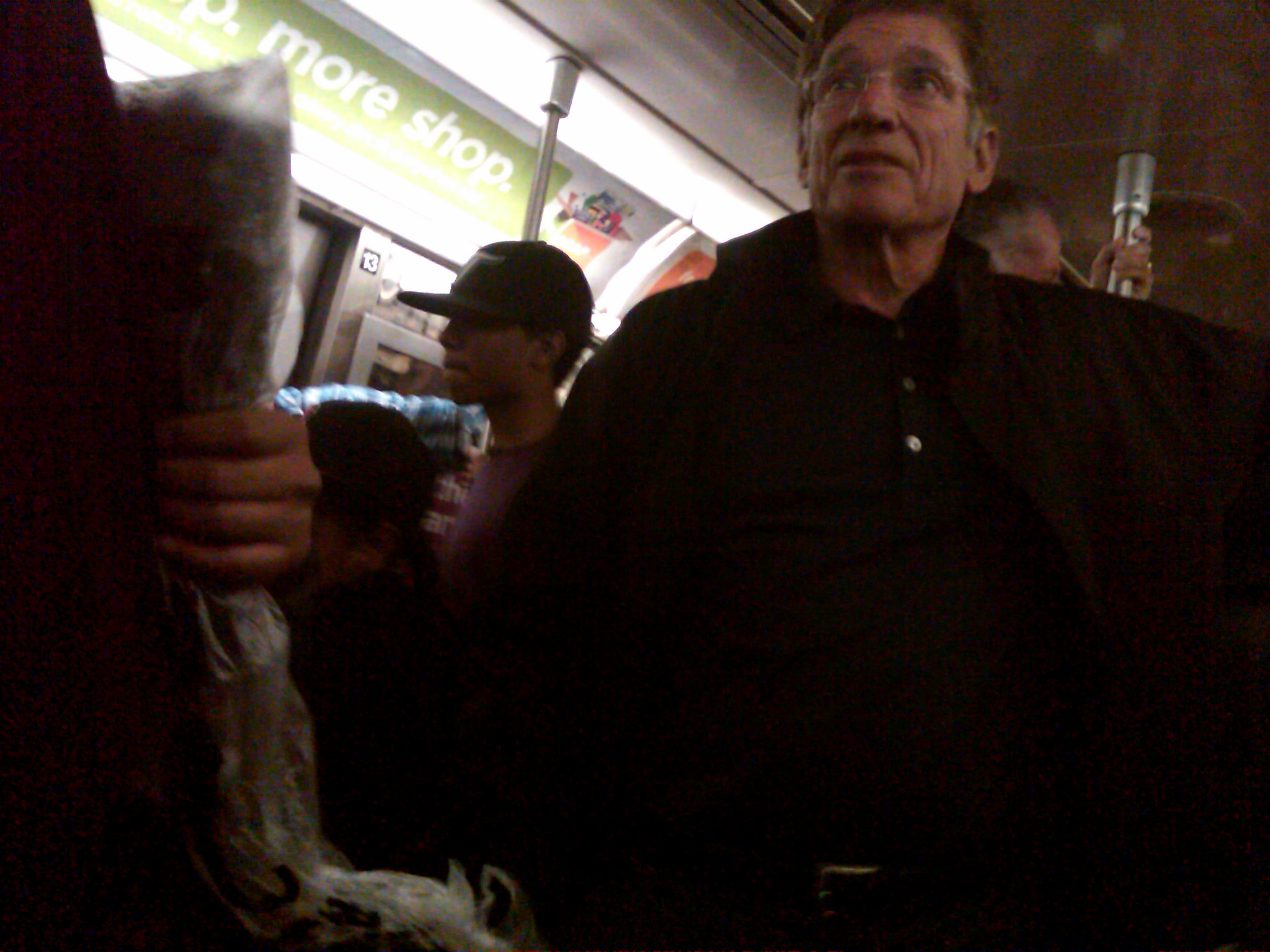The image captures a scene inside a dark subway car. At the forefront is an older gentleman, possibly in his 50s or 60s, who appears nervous and concerned. He wears thin glasses and is dressed in a black coat over a black shirt with a few buttons undone, revealing his belt. To his left stands a boy or young man in a baseball hat and a red shirt. Behind the older man, another individual is holding onto a pole and looking towards the right side of the frame. In the background, another person is visible, also grasping a pole. On the left side of the image, a hand is holding onto something, and a subway car door is slightly visible. Additionally, an advertisement with a green background and various icons is displayed inside the car.